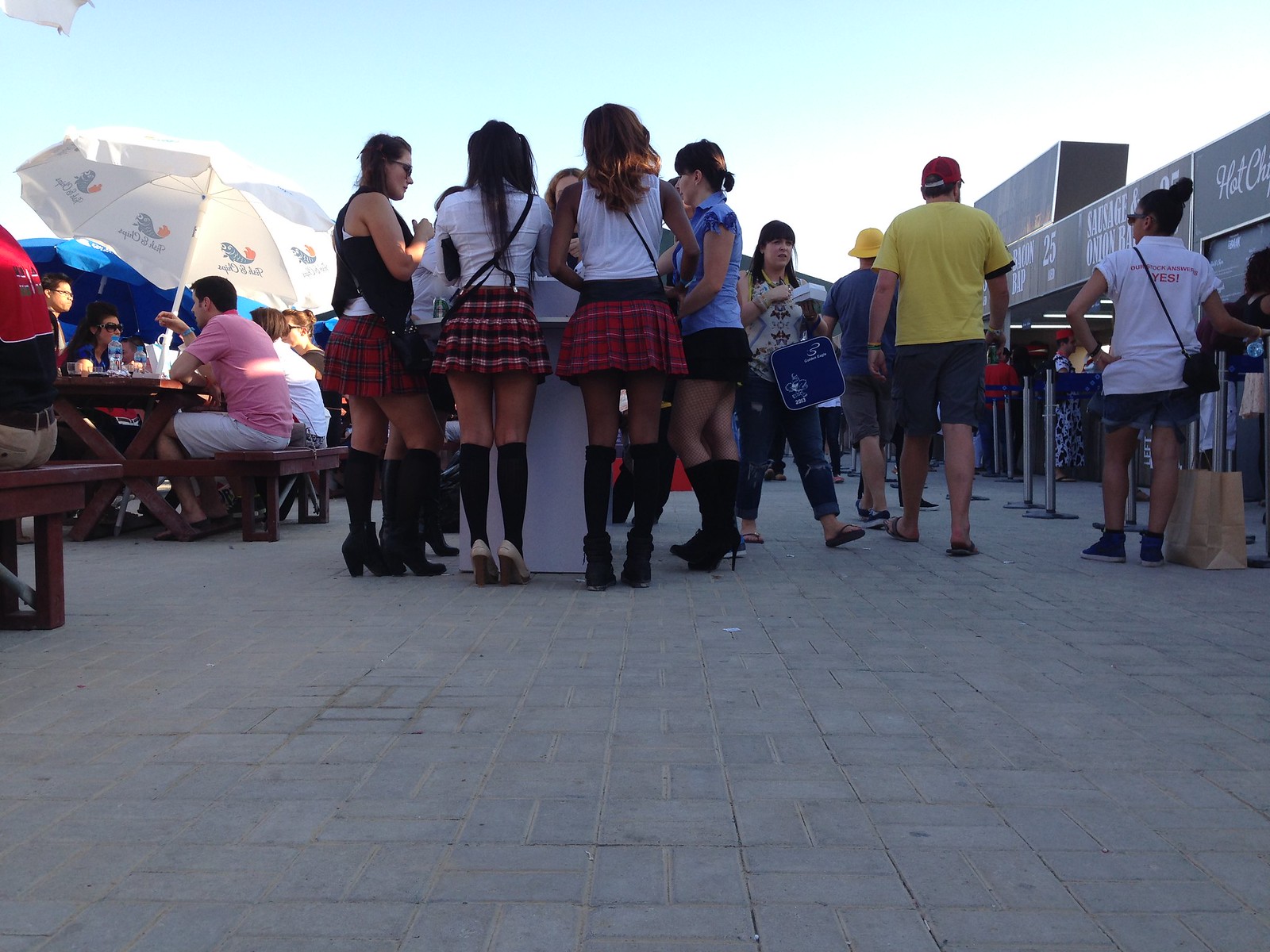The image depicts a bustling outdoor food market or fair filled with people enjoying various food options. On the right side, multiple food stands can be seen, including ones labeled "Hot Chips" and "Sausage and Onion Rings," with one stand's sign partially visible but unclear. Several people are seen waiting in lines at these vendors. In the center, a group of women stands around a white fixture, which could be a hand-washing sink or a table. These women are dressed similarly in red plaid skirts with matching tops, and they are wearing heeled boots or shoes. To the left, there are brown tables with blue and white umbrellas, where people are seated, eating, and drinking. The image is taken from a lower angle, giving a very detailed view of the scene and focusing on the activities taking place at this lively gathering.